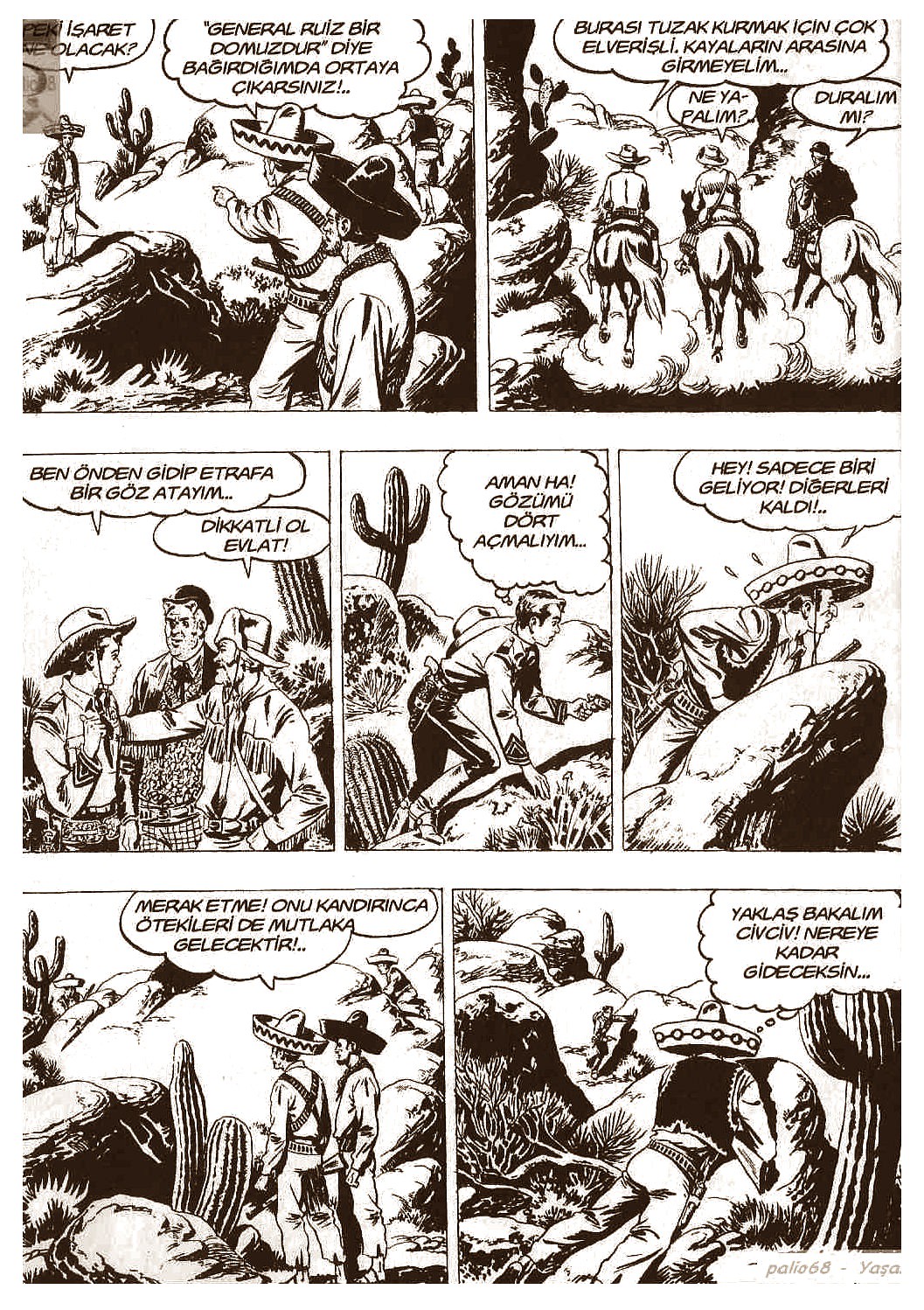This image is a scanned black and white comic strip featuring seven panels, laid out in three rows: two panels in the top row, three in the middle, and two in the bottom. In the top left panel, several characters, likely Mexican gunslingers wearing sombreros, are engaged in a conversation in a desert setting. The top right panel depicts three characters on horseback, riding away. The middle row begins with three men conversing next to a saguaro cactus, followed by one character sneaking away, and ends with another character watching from a rocky ledge. In the bottom row, two individuals are seen discussing something while others climb rocks, and the final panel again shows the man on the rocky outcrop observing the scene below. The comic dialogue is in a language other than English, and a small caption in the bottom right corner reads "Palio 68 Yasa."